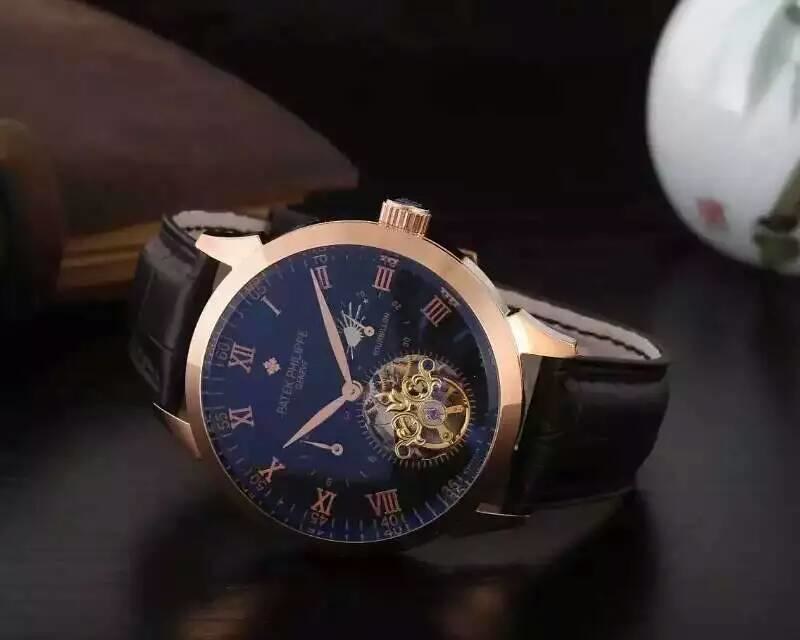This photograph, potentially an online store product image, captures a beautifully detailed wristwatch set against a dark, glossy background. The watch, prominently centered, features a rich brown leather band with stitched edges. Its face is a striking navy blue surrounded by a bronze-colored, metallic frame. The hands of the watch are also bronze, matching the frame. Roman numerals mark the hours and a distinctive small round window at the bottom of the watch face reveals intricate inner workings. The watch is slightly laying on its left side, providing a clear view of its elegant details. A gold dial adorns the top, complementing the bronze elements. To the upper right corner, a round white object is visible, while to the left-hand corner, a gold case, presumably for the watch, subtly appears. The watch’s reflection is visible on the dark, shiny surface, adding depth and dimension to the image.